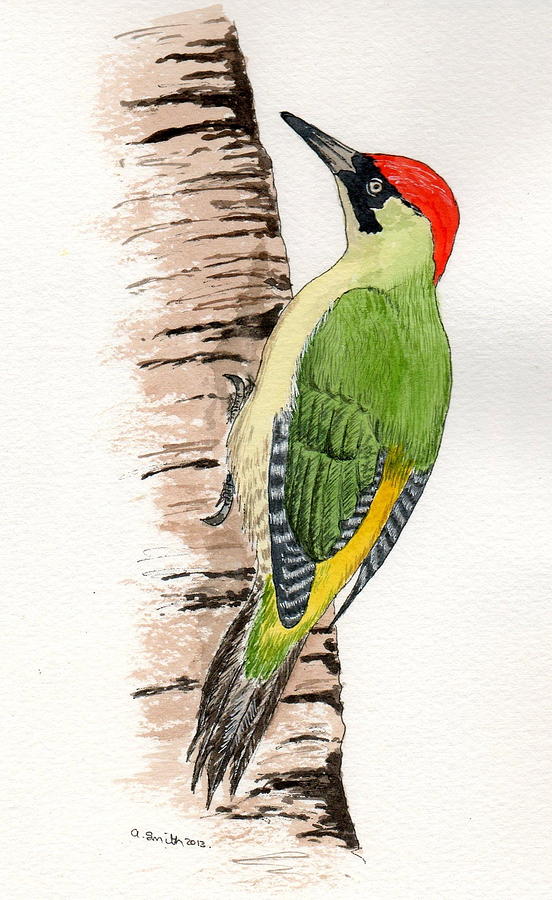The illustration depicts a woodpecker perched on the side of a light brown tree trunk with black shades. The woodpecker features predominantly green feathers with a hint of yellow on its body. Its back and wing tips display black and white stripes, while its underbody is a lighter green with cream and brown specks. The bird's head is crowned with a striking red crest, and it has a black face mask surrounding its eyes. The woodpecker's long, sharp gray beak is slightly open. The background of the drawing is a uniform gray, enhancing the bird's vibrant colors. The artist's signature is visible in black ink at the bottom left of the image, though it is too small to decipher. The illustration is rendered in colored pencil and captures the essence of ornithological art.